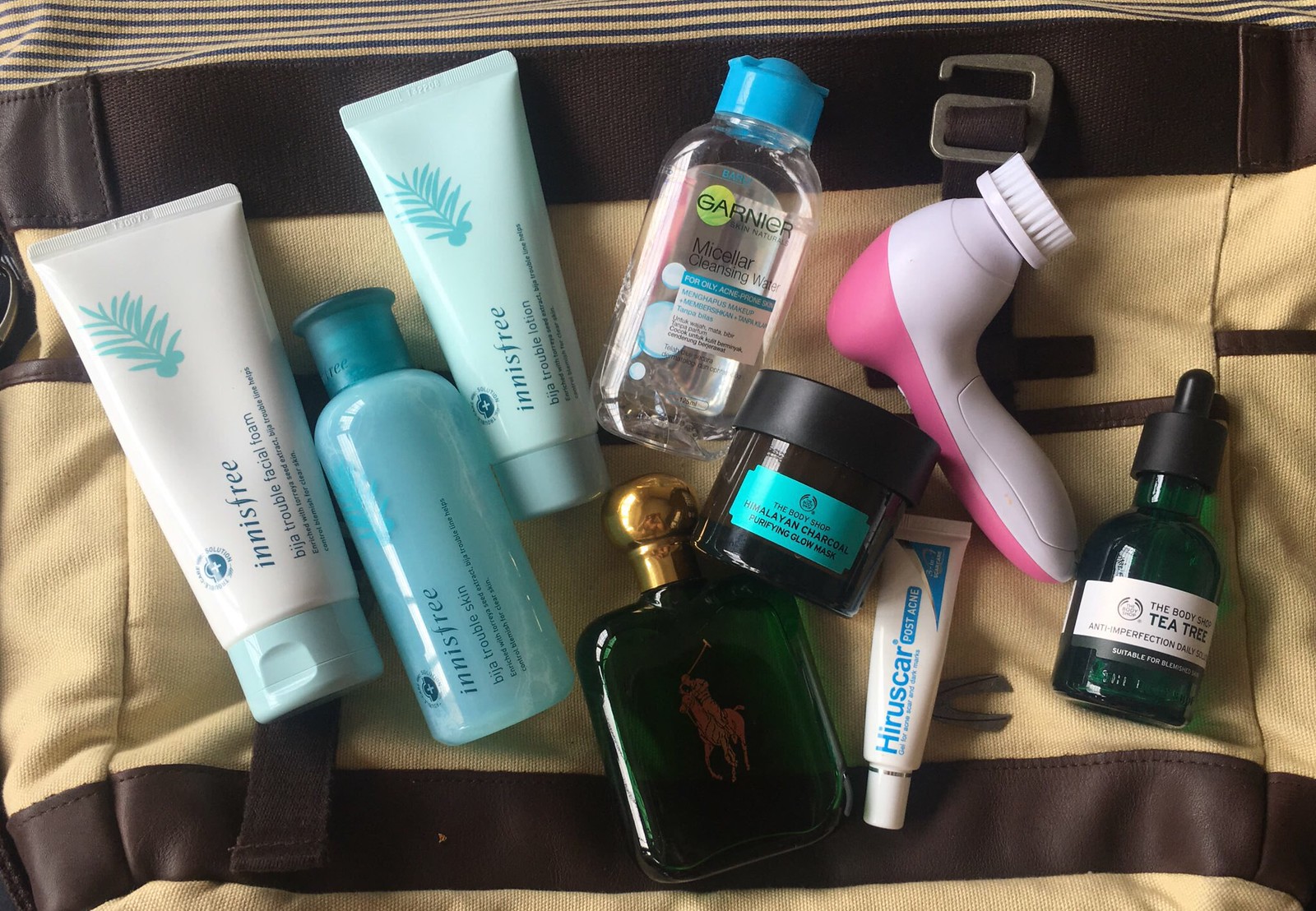This detailed image captures a meticulously organized collection of skincare and grooming essentials, all laid out presumably to be packed into the grey luggage bag in the background. Prominently displayed among the items are three products from the Innisfree line: a bottle of Innisfree Facial Foam with writing that appears to be in another language, Innisfree Trouble Skin toner, and an Innisfree lotion formulated for troubled skin. Additionally, a bottle of Garnier Micellar Water can be seen, essential for gentle cleansing. Complementing these are skincare treatments including Hero Scar Post Acne, a likely treatment for post-acne scars, and a luxurious small jar of Himalayan Charcoal Purifying Glow Mask from The Body Shop. There’s a touch of fragrance with a sleek bottle of cologne, while a pink spinning facial brush with bristles speaks to a high level of skincare routine. Completing the array is The Body Shop's Tea Tree Anti-Perfection Daily solution, housed in a dropper bottle, although the full name is slightly cut off in the image's view. The careful arrangement of these items suggests a well-planned packing strategy for a traveler committed to a comprehensive beauty regimen.